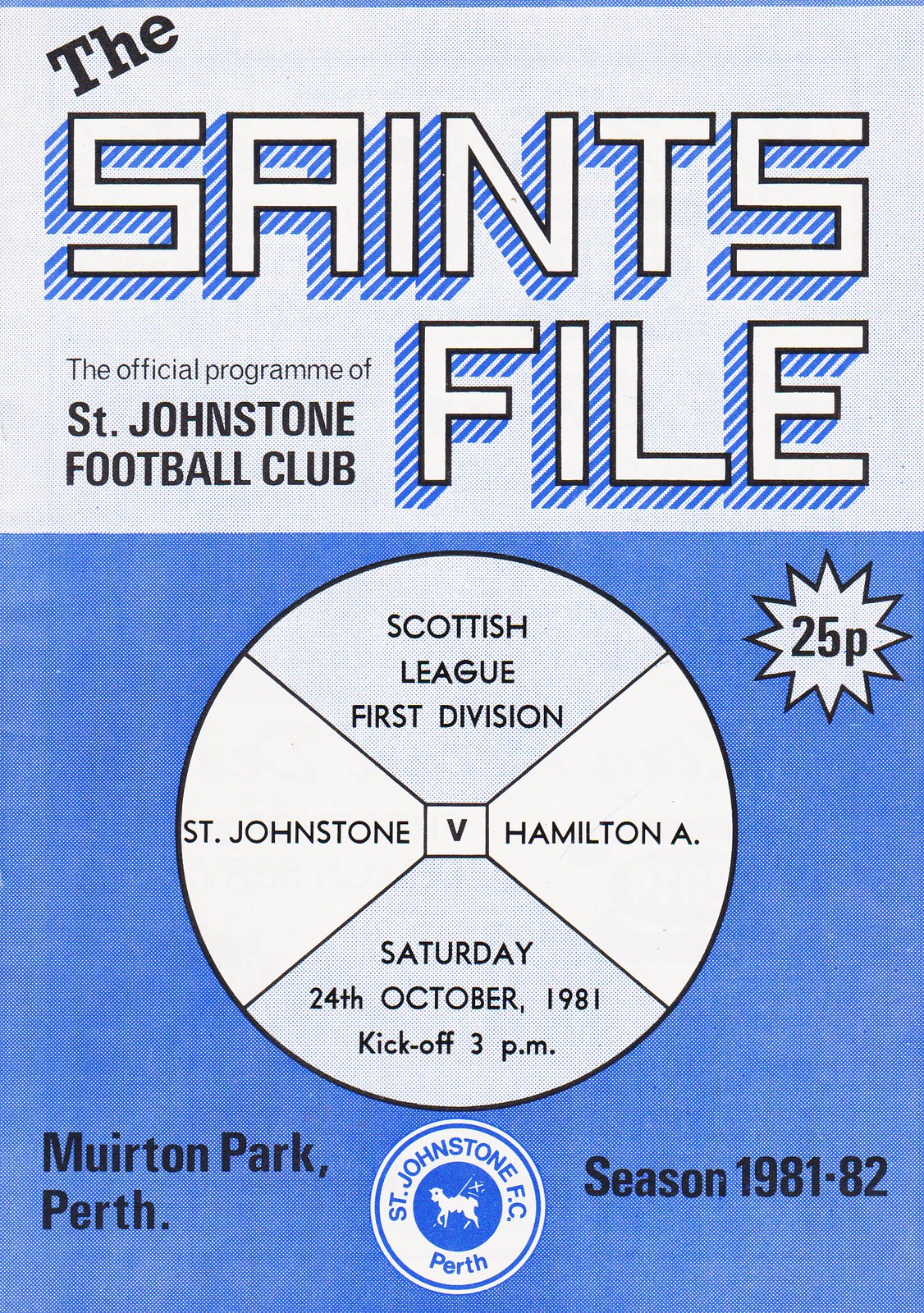The image is a scan of the cover for a football program, specifically for St. Johnstone Football Club. The layout is split between white and blue sections. In the top left corner of the white section, black text reads "The," followed by "Saints File" in white text with a black border. The bottom left corner of this white section designates the document as the official program of St. Johnstone Football Club. Transitioning to the blue section at the bottom, a starburst graphic in the top right corner indicates the price of 25p. Central to this section is a circular diagram divided into four segments, with "Scottish League First Division" at the top, "Hamilton A" on the right, "St. Johnstone" on the left, and "Saturday, 24th October 1981, kickoff 3 PM" at the bottom. At the very top and bottom of the cover, additional text mentions "Merton Park, Perth" and "season 1981-82." Finally, a logo at the bottom, featuring a lamb carrying a flag, represents St. Johnstone FC Perth. The overall design is simple and uses a color scheme of whites, blacks, and blues, with no photographs of people.